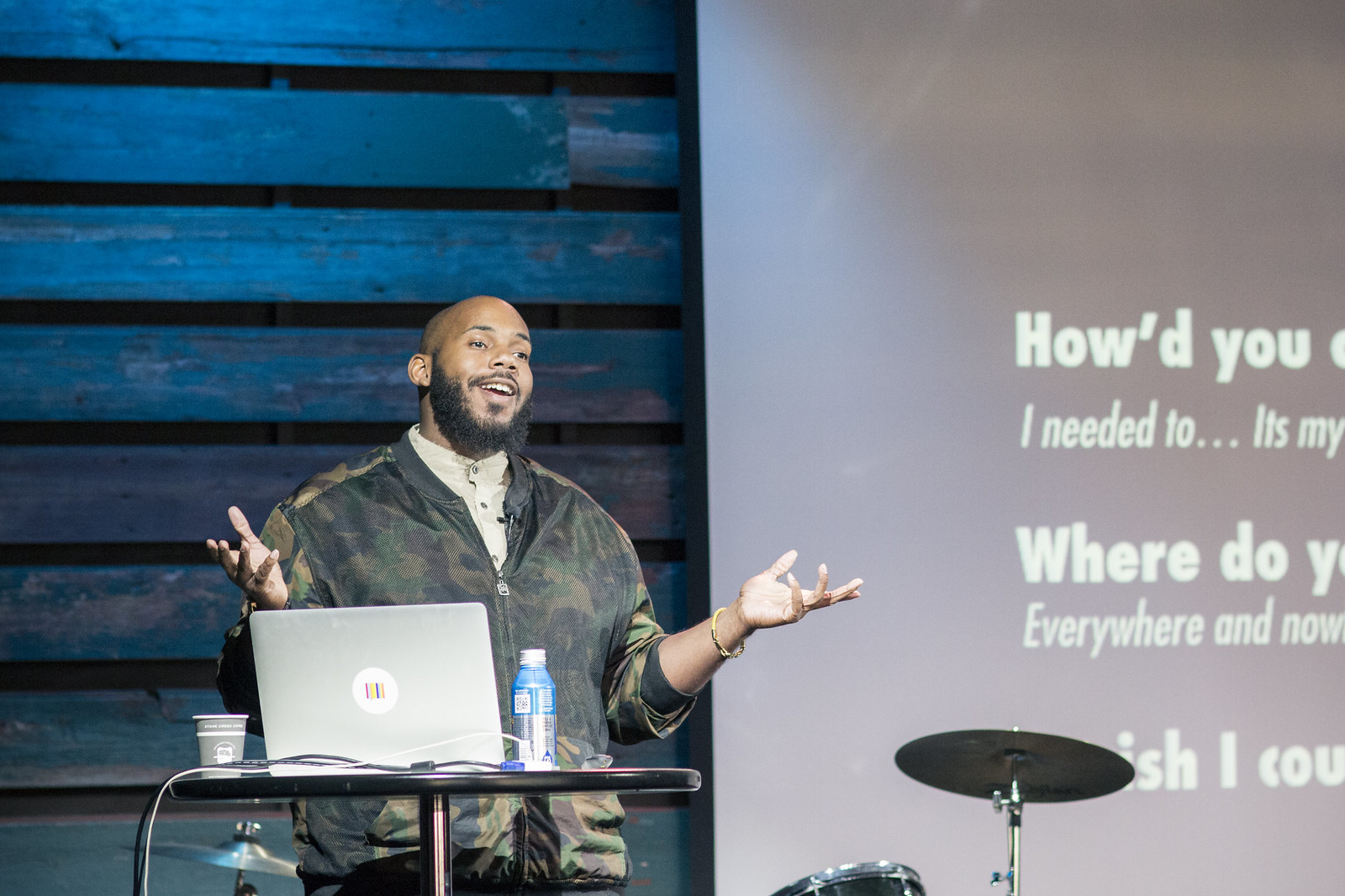In this detailed indoor scene from a presentation, a black man with a bald head and facial hair stands confidently on stage. He is positioned in front of a podium adorned with a silver laptop, a bottle with a blue cap and blue and silver label, and a paper coffee cup. He wears a camouflage bomber jacket over a buttoned shirt, and his hands are extended upward to chest level, palms open, conveying engagement with his audience. Behind him is a striking backdrop of wooden slat panels illuminated in blue, partially giving way to a large projection screen. Text on the screen, though partially obscured, reads lines such as "how do you," "I needed to," and "it's my," suggesting the posing of reflective questions. Further adding to the layered setting, a cymbal from a drum set is visible on the lower right portion of the image, hinting at the presence of musical equipment in the vicinity.